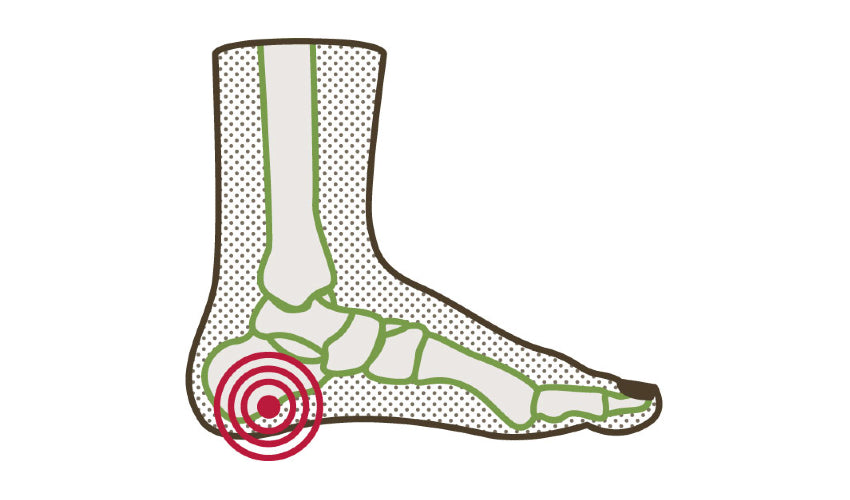The detailed, unified caption for the image could be:

This color illustration, presented in landscape orientation against a white background, depicts an internal view of a person's left foot from just above the ankle to the toes. The bone structure, outlined in dark green, is prominently featured, with a light gray interior. The single visible big toe extends to the right, while the calcaneus (heel bone) is located on the left. Surrounding the calcaneus are distinct red concentric circles forming a target, possibly indicating an issue such as plantar fasciitis. The foot itself is overlaid with a translucent greenish pattern and green polka dots, reminiscent of a see-through boot. The drawing highlights the interconnected bones of the foot - including the tibia, tarsals, and metatarsals - suggesting a clinical focus on the highlighted area at the heel.